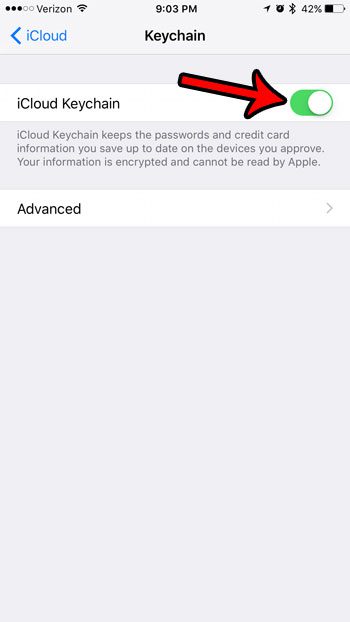This detailed caption describes a screenshot from an iPhone displaying the iCloud Keychain settings page.

---

The screenshot captures the display of an iPhone at 9:03 PM, connected to Verizon with a Wi-Fi connection, and showing a 42% battery life along with active location, timer, and Bluetooth symbols. At the top left, three out of five dots are filled, indicating the current screen in a sequence. The main content shows the iCloud Keychain settings page, with bold black text at the top reading "Keychain." A blue "iCloud" text with a left-pointing arrow is displayed on the top left, indicating navigation back to the previous iCloud settings page. Below, there's an "iCloud Keychain" option highlighted by an active green toggle switch on the right. Additional information under the toggle explains that iCloud Keychain keeps passwords and credit card information up to date across approved devices, with all information encrypted and unreadable by Apple. At the bottom, there's an "Advanced" option with a right-pointing arrow, suggesting further settings available but not currently expanded.